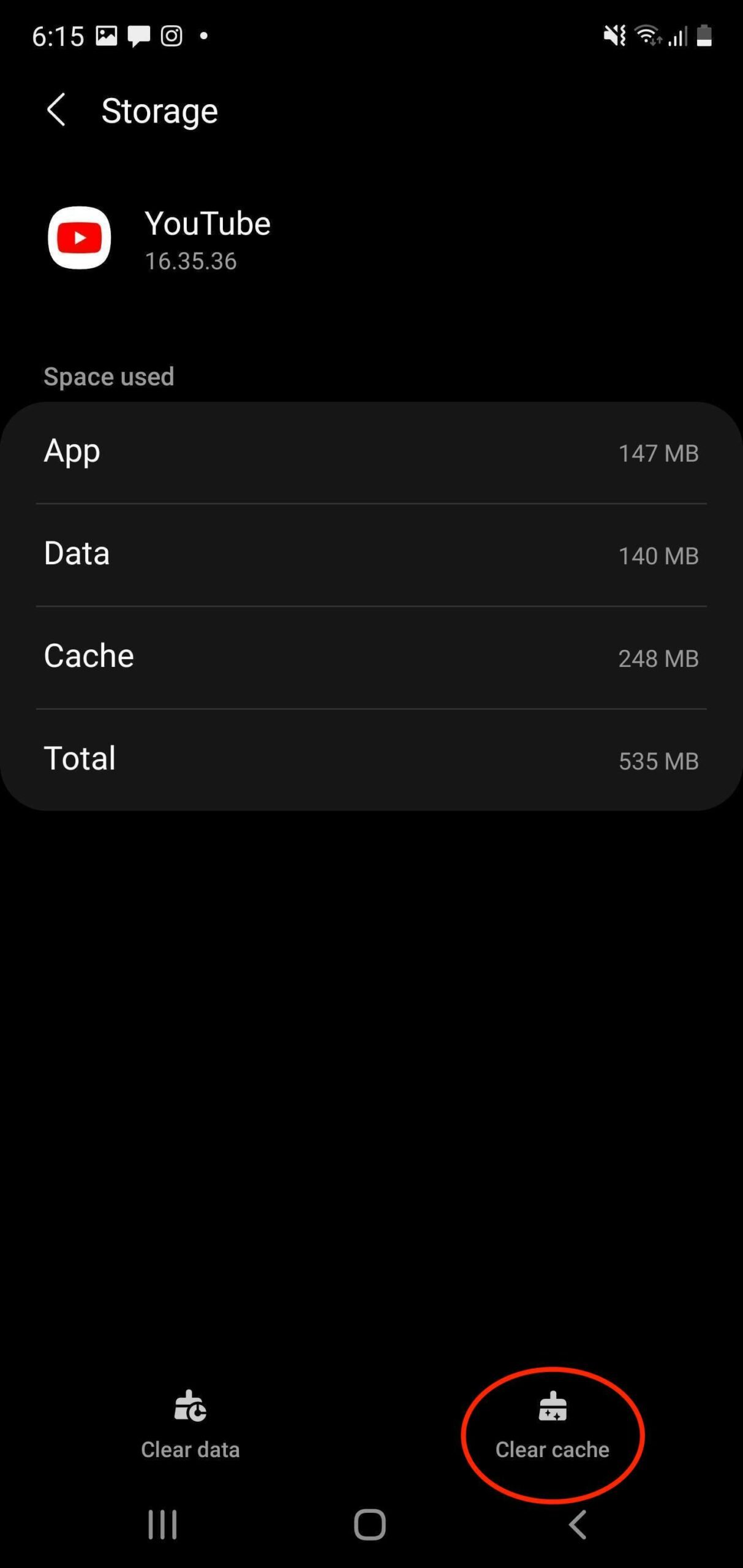Screenshot captured at 6:15 PM displaying the storage settings for the YouTube app on a smartphone. The status bar at the top shows various icons indicating a battery level at approximately 20%, 3 out of 4 bars for signal strength, active Wi-Fi, and notifications. The phone is currently on the storage information screen for YouTube version 16.35.36, detailing the space used. The space usage is broken down as follows: the app itself takes up 147 megabytes, user data occupies 140 megabytes, and cached data consumes 248 megabytes, making a total of 535 megabytes. Below this table are two actionable icons labeled "Clear data" and "Clear cache," with the latter highlighted by a prominent red oval. Further down, three additional icons are visible: a grid icon with three vertical bars, a rounded square, and a left-pointing arrow. The entire interface has a black background, enhancing the readability of the text and icons.